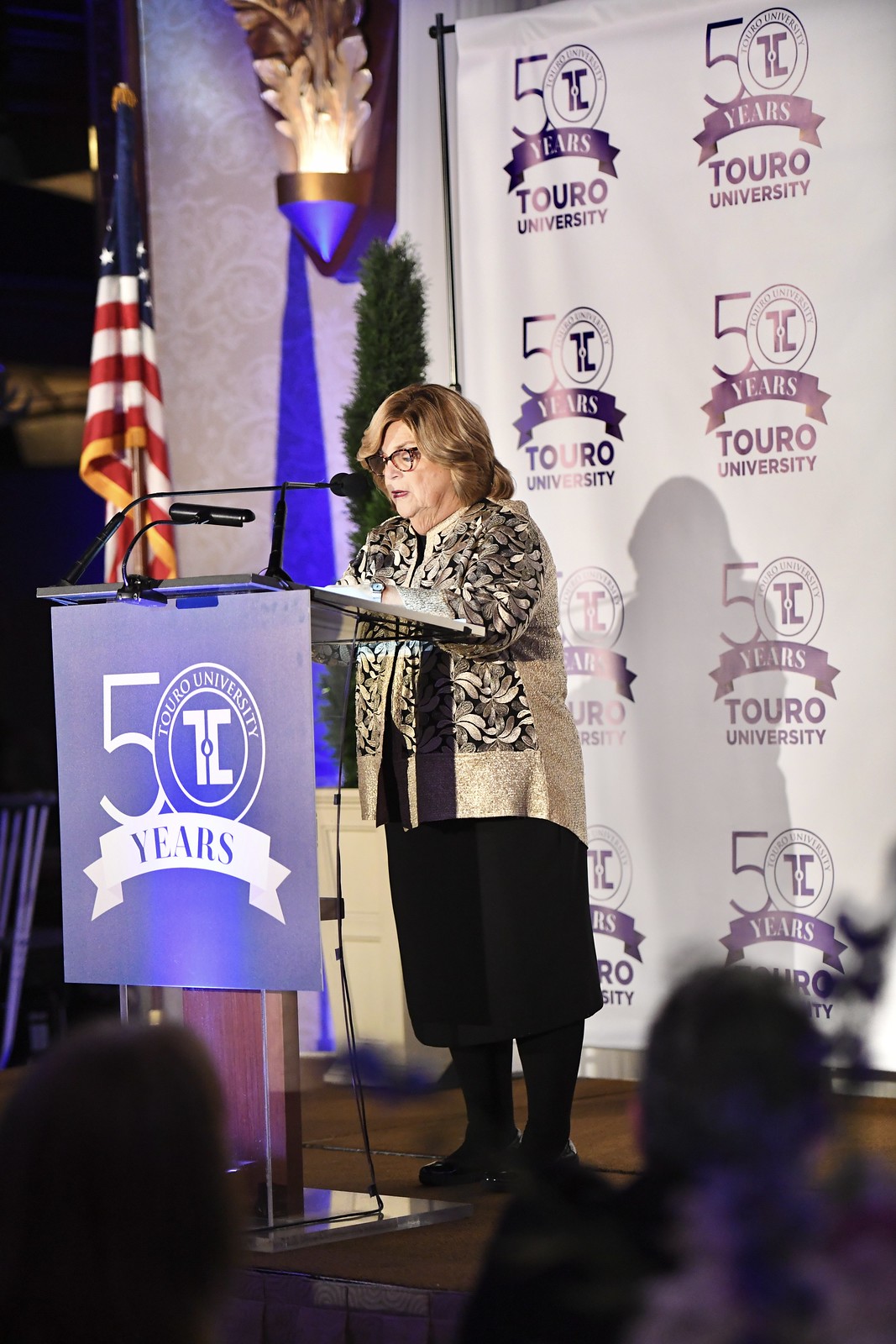An older woman with short blonde hair and glasses is standing at a wooden podium on a stage, delivering a speech into a black microphone. The podium features a dark blue display with white text that reads "50 years, Touro University" with the "0" designed as a donut shape with a blue center. She is dressed in a golden-brown and blue sweater-like top, a black skirt, black leggings, and black shoes. Behind her is a white backdrop repeating the "50 years, Touro University" logo with blue ribbons, creating a celebratory atmosphere. An American flag and a potted plant are also visible on the stage, and the audience, whose faces are not clearly seen, appears engaged, suggested by a few visible hands and attentive posture. The backdrop is brightly lit, casting blue shadows and enhancing the festive setting of the award ceremony. The woman speaks with a slight grin, indicating a positive and engaging presentation.